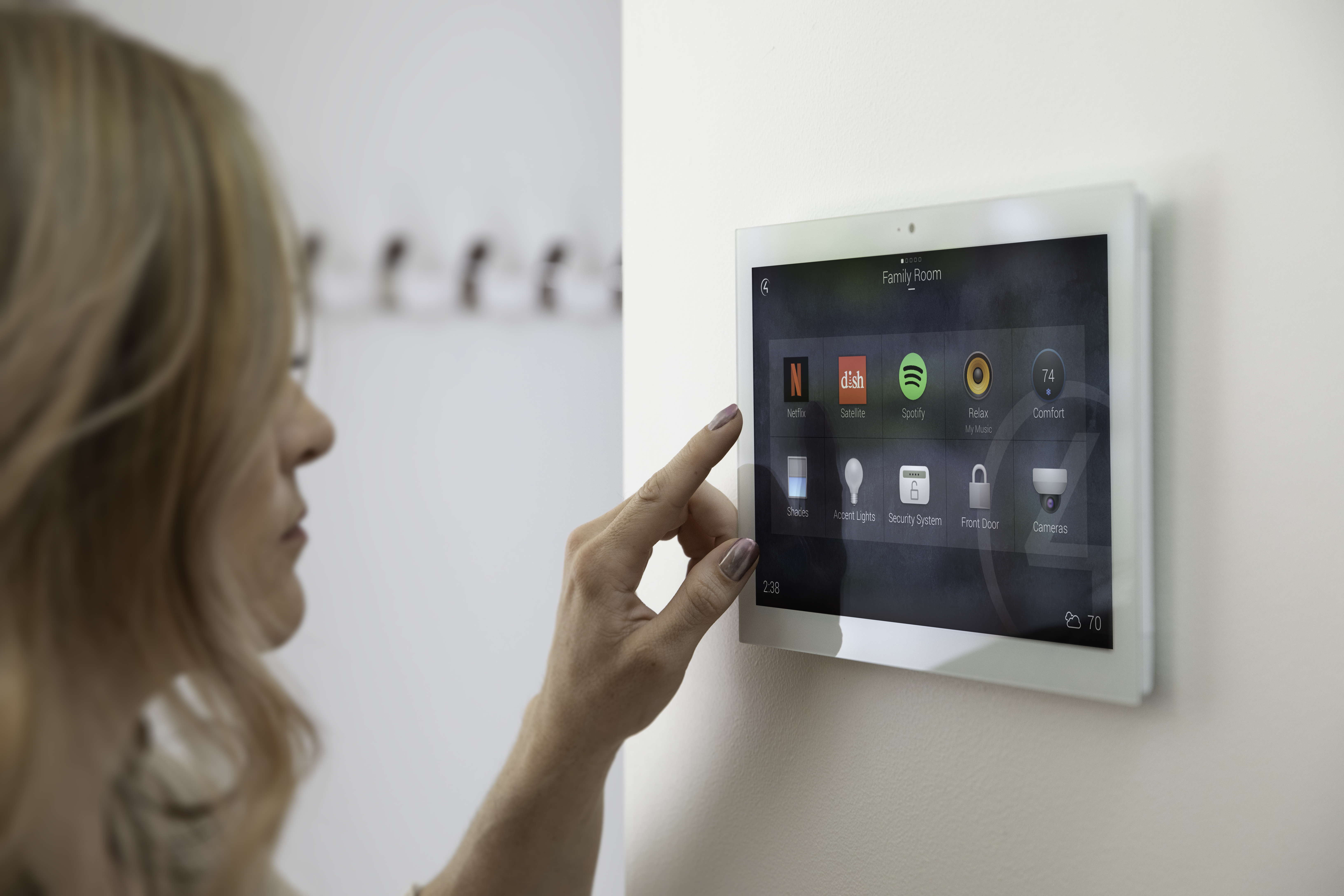In this image, a woman is seen standing to the left, poised to interact with a smart home control panel, which is designed similarly to a tablet, mounted on a white wall. The device features a black screen with a white border, displaying an array of app icons arranged in two rows. Among the icons, Netflix is positioned in the top left corner, with other visible icons including Spotify, Dish, a lock symbol for security, and one labeled "cameras." The smart panel is labeled "family room" at the top, suggesting it monitors and controls various aspects of the house. The woman, who has nail polish on her extended left hand, appears to be about to tap the Netflix icon. The tablet also displays the time, temperature, and weather, integrating multiple smart home functions into a sleek interface.